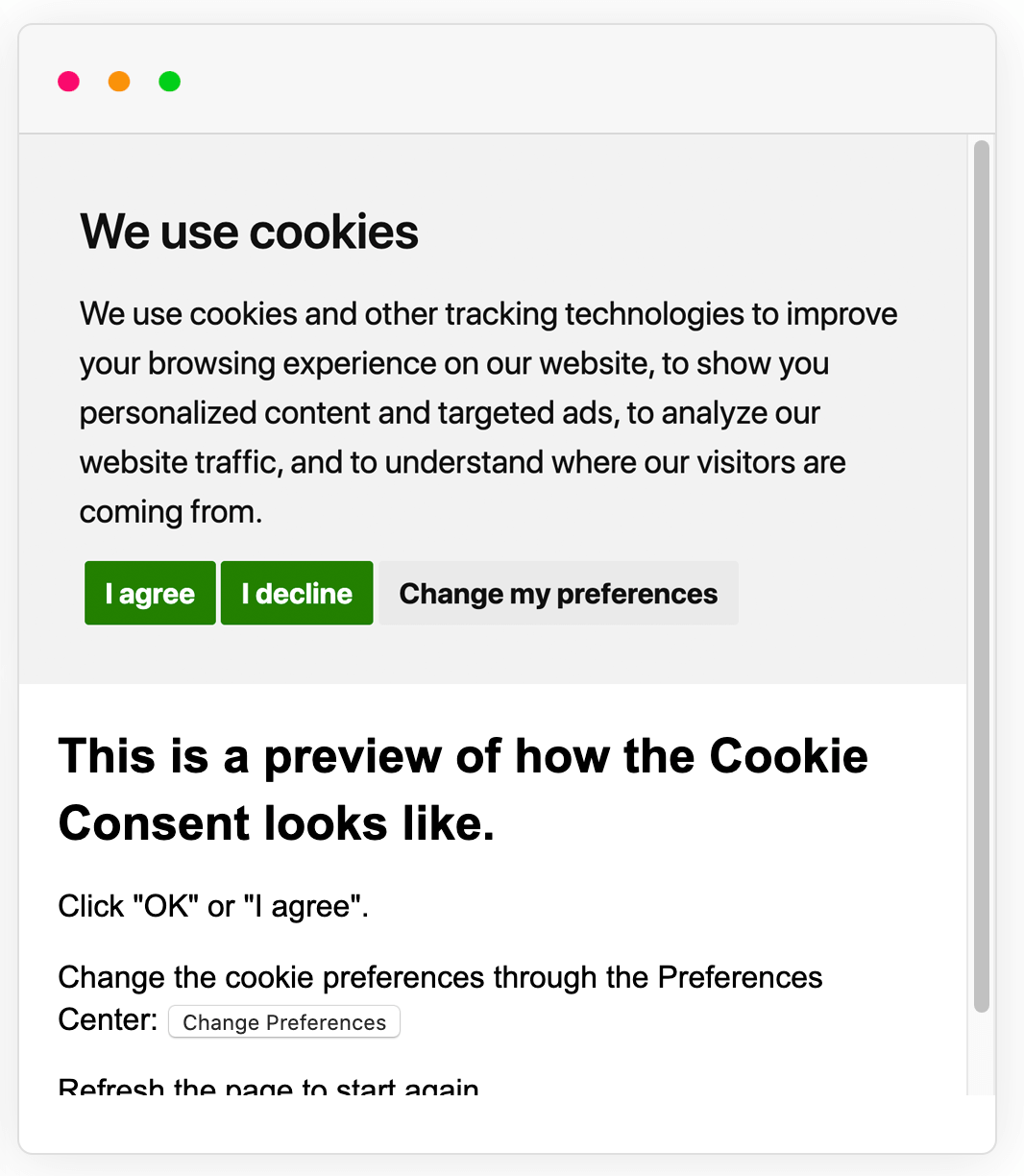The image displays a cookie consent notice with a two-toned background: the top half is light grey, and the bottom half is white. Centered on the light grey section, black text reads: “We use cookies and other tracking technologies to improve your browsing experience on our website, to show you personalized content and targeted ads, to analyze our website traffic, and to understand where our visitors are coming from.” 

Below this text, three buttons are aligned horizontally. The "I Agree" and "I Decline" buttons are green with white text, while the "Change My Preference" button is grey with black text. The "Change My Preference" button is positioned to the right.

In the white lower half of the image, additional black text states: “This is a preview of how the cookie content looks like. Click OK, or I agree. Change the cookie preference through the preferences center. Change preferences.” The “Change preferences” text is set in a slightly grey rectangular button, signifying it as an interactive element. Another line of text below reads: “Refresh the page to start again.”

On the right side of the image, there is a grey vertical slider indicating the scroll functionality for the page.